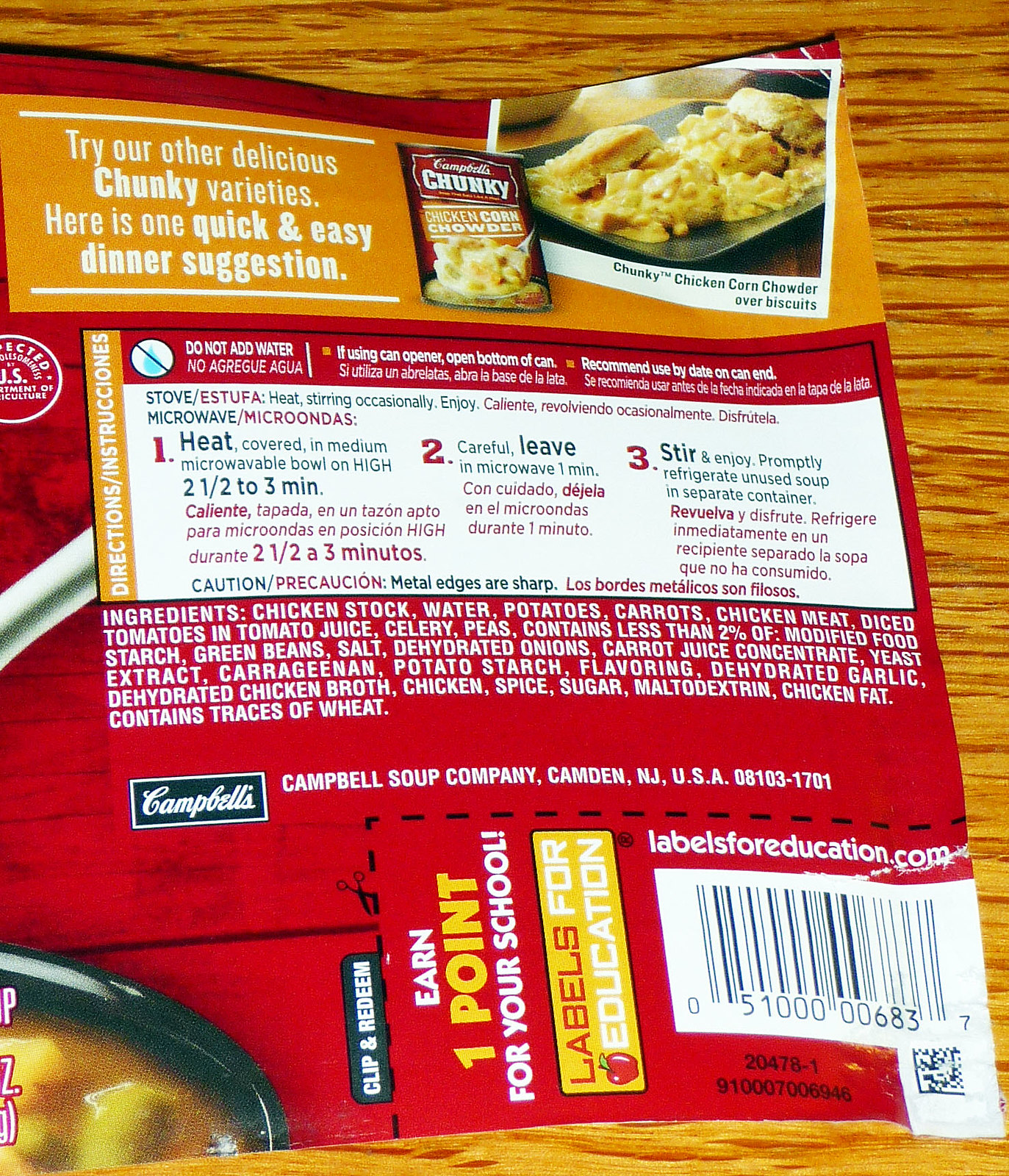This image features the backside of a label from a can of Campbell's Chunky Soup, carefully removed from the can and laid flat on a wooden tabletop. The label is predominantly dark red, creating a cohesive backdrop that frames the detailed information presented. The upper section of the label includes an orange stripe with the enticing message: "Try our other delicious Chunky varieties." This section also provides a quick and easy dinner suggestion, featuring a recipe for creating Chunky Chicken Corn Chowder over biscuits using the soup. Below the recipe suggestion lies a boxed section with clear instructions for microwave cooking. Further down, a comprehensive list of ingredients details the various contents of the soup. The overall presentation on a rustic wooden surface adds a homey and practical aesthetic to the informative label.